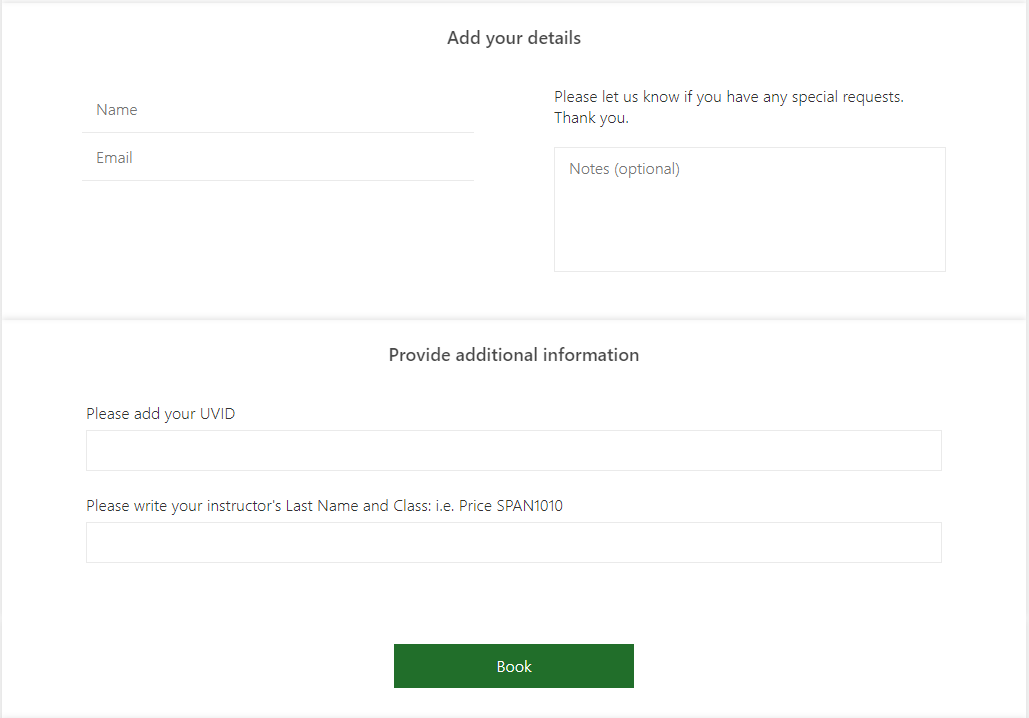This screenshot features a web page designed as a fill-in form with two distinct sections. 

The first section, centrally titled "Add Your Details," contains fields on the left side for user's personal information. These fields include "Name" and "Email," each with a line underneath where users can input their information. On the right side of this section, there's a prompt reading "Please let us know if you have any special requests. Thank you." Below this prompt, there is a text box labeled "Notes (Optional)" for users to provide any additional comments or requests.

The second section, titled "Provide Additional Information," consists of further input fields. On the left side, there is a prompt asking users to "Please add your UV ID," accompanied by a text box for entering the ID. Below this, there's a prompt reading "Please write your instructor's last name and class, i.e., Price, SPAN 1010," with another text box for this information.

At the bottom center of the form is a green button labeled "Book," likely used to submit the form.

The overall design of the webpage is clean and minimalistic, with a predominantly white background and a light gray border enclosing the form. A horizontal line separates the two distinct sections. All text on the page is presented in dark shades of black or gray for clear readability. The headings are slightly larger in font size compared to the input labels, providing a clear visual hierarchy.